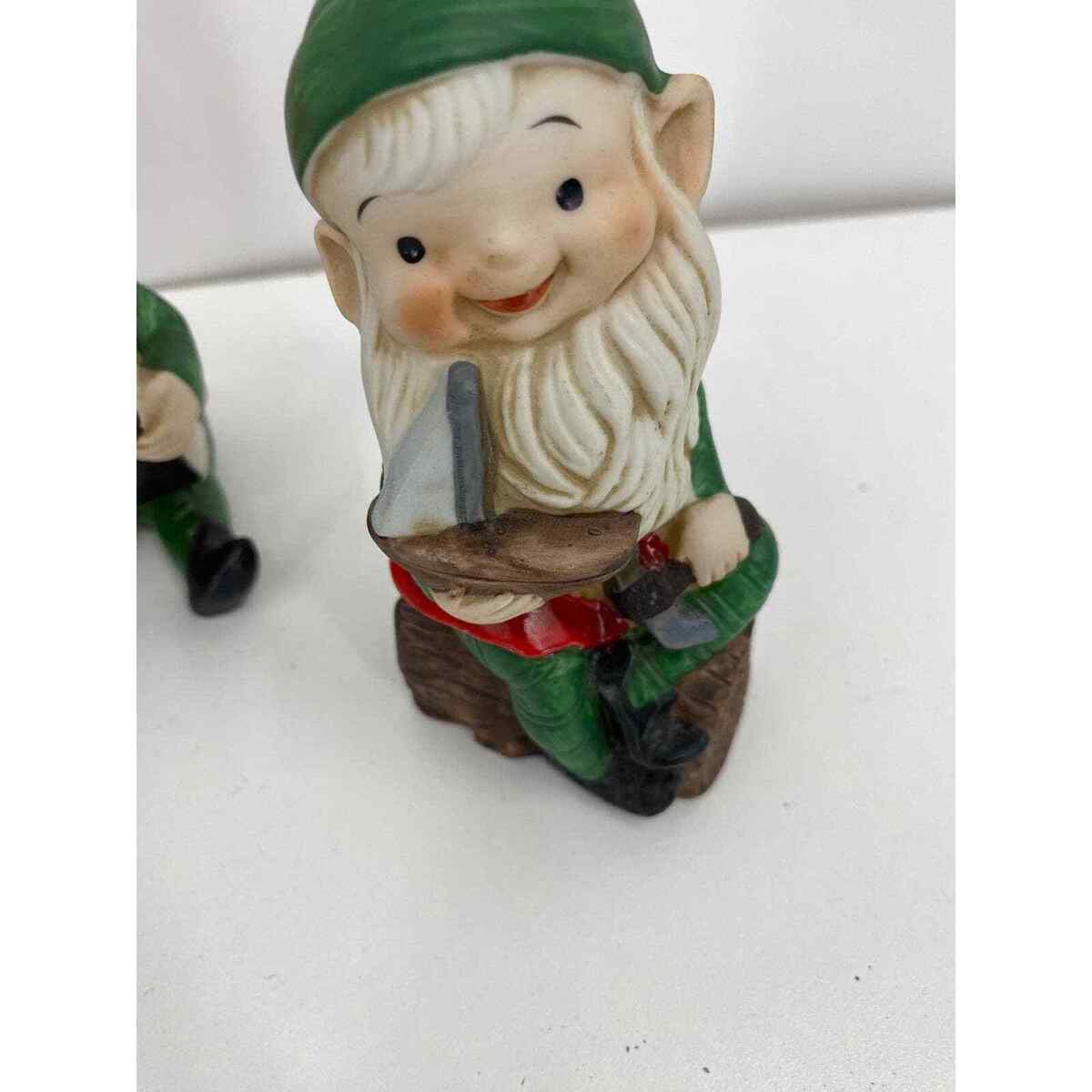This image depicts a detailed close-up of a collectible ceramic garden gnome, seated on a dark brown log. The background is stark white, providing contrast to the vibrantly colored figurine. The gnome is adorned in a dark green beanie or elf hat, though the top is slightly cropped out of the frame. It has white bangs peeking from under the hat and a long white beard with a cheerful face marked by beady black eyes, rosy red cheeks, and large ears. The gnome wears a long-sleeved green shirt, a red belt, long green pants, and black shoes. Clutched in its hands is a small toy boat, featuring a wooden hull, an off-white sail, and a gray mast. To the left of the gnome, partially visible, is another gnome marked by a black shoe, a green pant leg, and a green-sleeved arm, hinting at a whimsical scene beyond the primary figure.